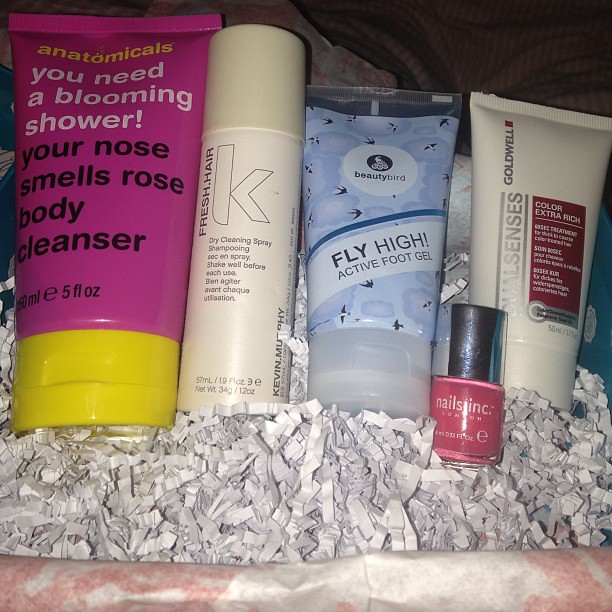This highly detailed color photograph captures five personal care items meticulously arranged inside a box lined with white filler paper, resembling confetti, for packaging protection. Starting from the left, there is a pink tube with a yellow cap labeled "Anatomicals: You Need a Blooming Shower, Your Nose Smells Rose Body Cleanser" with a volume of 5 fluid ounces. Next to it sits an off-white can of dry cleaning spray, marked "Fresh Hair" with a prominent 'K' and the instruction to shake well before use. In the center of the arrangement is a blue tube of "Beauty Bird Fly High Active Foot Gel," adorned with a cloud-like design. To its right is a small bottle of dark red nail polish with a black cap, branded "Nails Inc." Finally, on the far right, a white tube with a white cap, labeled "Goldwell Color Extra Rich," stands partially in the background. The items are clearly selected for a theme of personal grooming and care, presented in a secure and aesthetically pleasing manner.